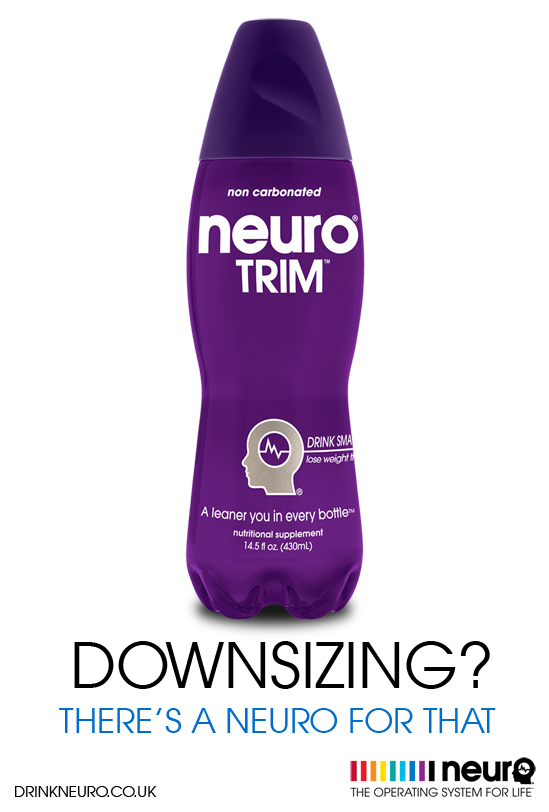The advertisement image displays a portrait-oriented product, featuring a beverage in a uniquely designed, plastic bottle reminiscent of a rocket or missile shape. The bottle is primarily a light purple-mauve color, accented by a darker purple, semi-triangular cap with a flat top and a notch to facilitate opening. The bottle's design includes curves that indent at the center and expand outward at the top and bottom.

Prominent white text at the top of the bottle reads "Non-carbonated Neuro Trim," with "Neuro" spelled N-E-U-R-O. Towards the mid-section, though curving slightly away, the text appears to state "Drink Smart. Lose Weight." Below this, additional text proclaims, "A leaner you in every bottle, nutritional supplement." 

Beneath the bottle, on a plain white background, black text asks, "Downsizing?" followed by blue text asserting, "There's a Neuro for that." In the bottom left corner, the website "drinkneuro.co.uk" is displayed. Near the right side of the image is an illustration featuring a colored rainbow emblem and the phrase "The operating system for life" in black text beneath the word "Neuro."